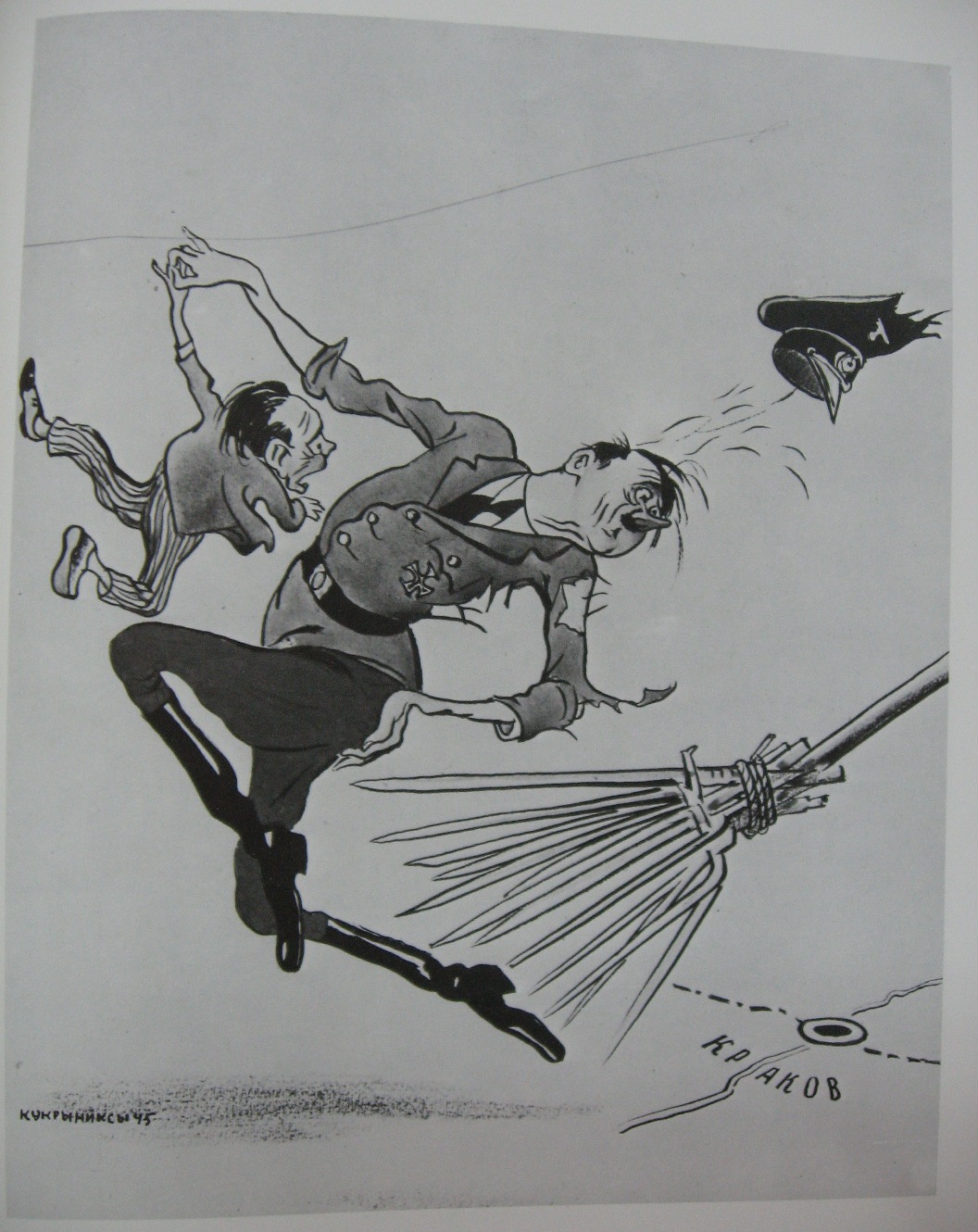The image is a black and white caricature drawing, resembling a political cartoon. At the center, a figure dressed in a Nazi uniform, unmistakably similar to Hitler with his characteristic mustache, is depicted. Hitler is being swept off the ground by a sharp, sword-like broom that has struck him painfully in the backside, causing him to leap into the air. His military hat is shown flying off his head. In his right hand, Hitler is clutching a much smaller man, roughly a third of his size, who is also caught in the airborne tumble. The smaller man appears to be depicted as similarly affected by the broom's strike. Below the scene, the ground features a map with what looks like crossroads and Russian text; notably, the text includes "K P A K O B," potentially a signature or notation, indicating possibly a Russian context or artist.